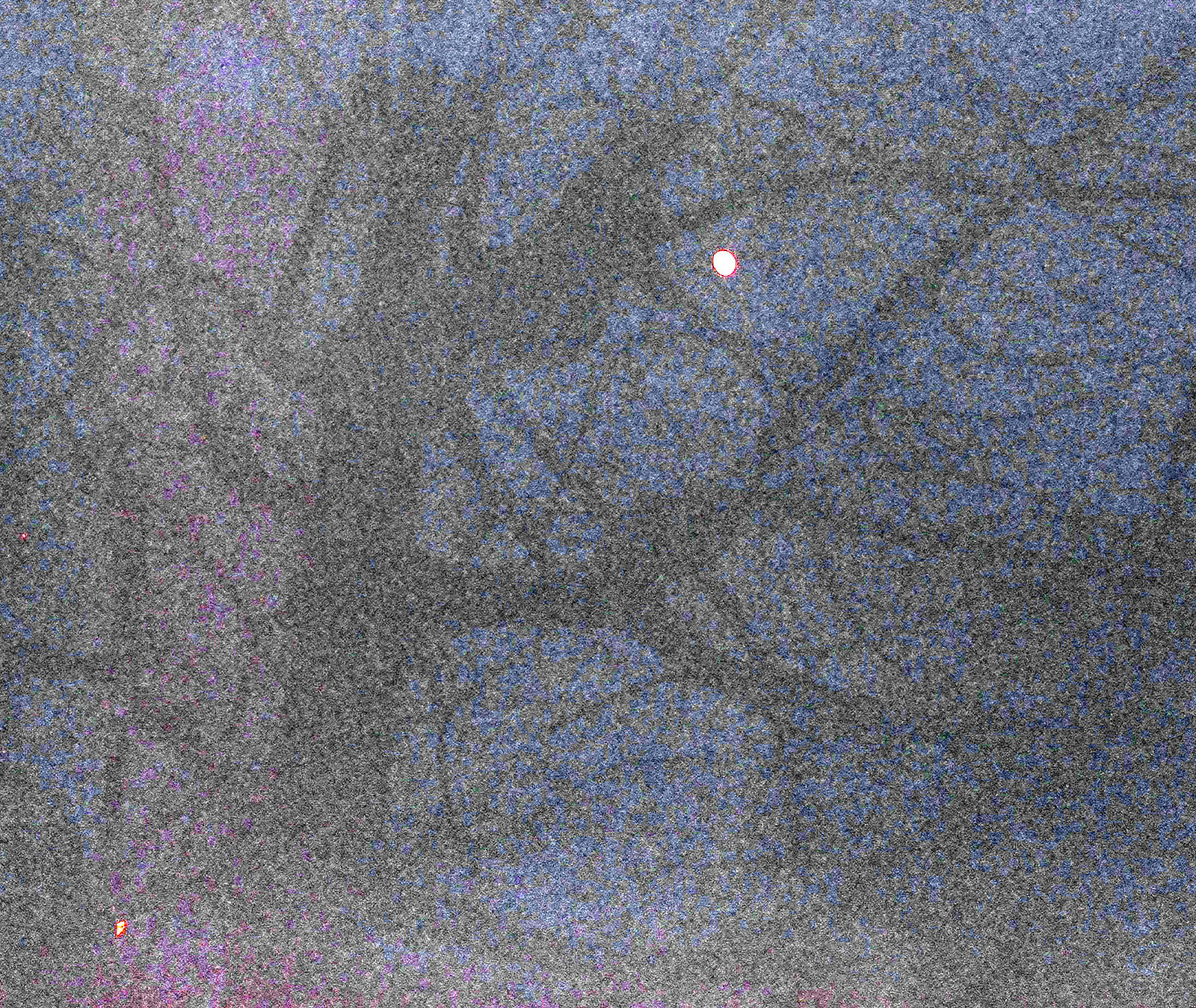Despite its grainy quality, this landscape-oriented photograph captures a hauntingly beautiful scene. Almost square in dimensions but not quite, the image looks out towards a bare tree, its intricate network of branches starkly outlined against the sky. The moon, faint but luminous, hangs in the background, adding an ethereal glow to the twilight scene. The sky itself transitions from a soft, dusky blue to a hint of purple on the left-hand side, creating a subtle gradient that enhances the composition. Though grainy, the texture adds to the eerie, almost vintage ambiance of the photograph, capturing the quiet, contemplative mood of this leafless tree silhouetted against the evening sky.